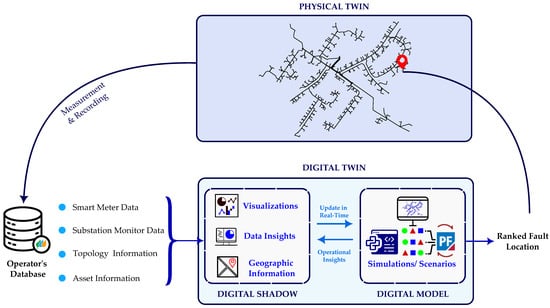This image depicts a detailed diagram on a white background, primarily using light blue and navy blue colors. The top section is labeled "Physical Twin" and features a blue rectangle filled with complex, interconnected lines resembling a family tree. This section includes a red location pin labeled "Ranked Fault Location." An arrow labeled "Measurement and Recording" extends from the left side of the physical twin box to a cylinder labeled "Operator's Database," which is further detailed with bullet points: "Smart Meter Data," "Substation Monitor Data," "Topology Information," and "Asset Information."

Below the physical twin is a second blue rectangle labeled "Digital Twin." This section includes several components such as "Visualizations," "Data Insights," "Geographic Information," "Digital Shadow," and "Digital Model." Additionally, it mentions "Simulation Scenarios" that contribute to operational insights. The entire diagram illustrates the relationship and data flow between the physical and digital twins, showcasing how measurements and recordings from the physical twin are processed and utilized within the digital twin to provide real-time updates and scenario simulations.